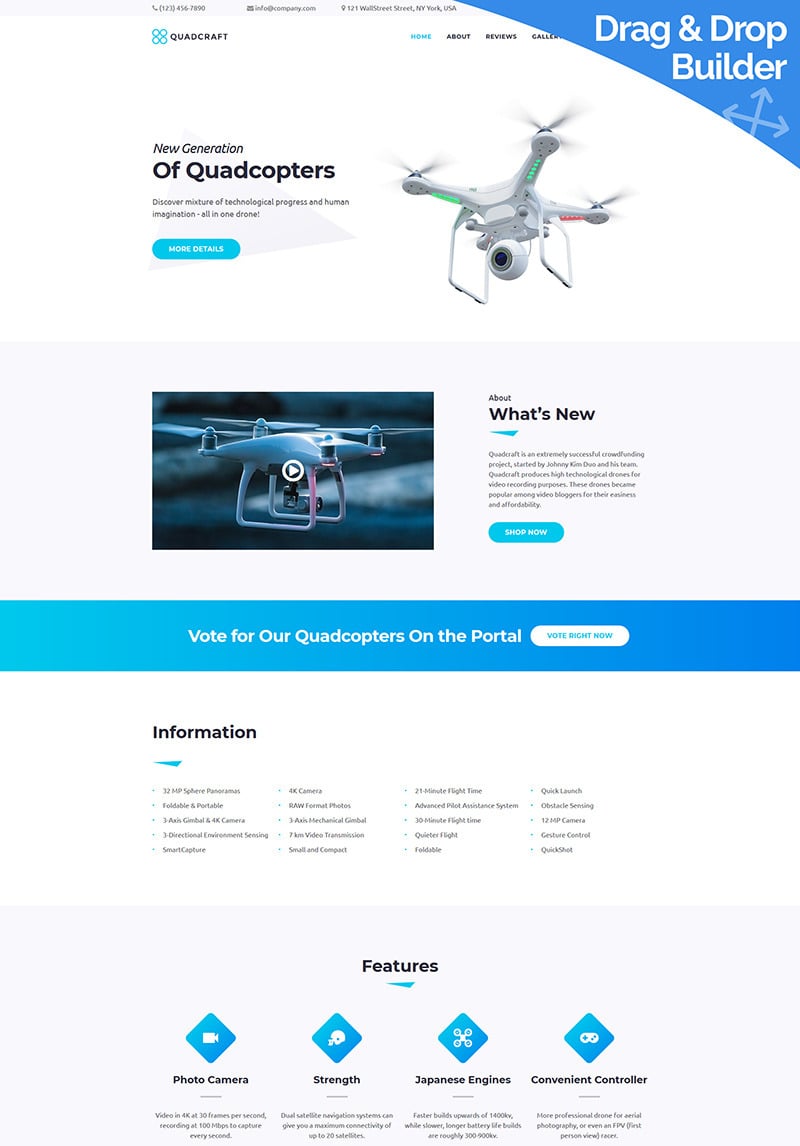The image appears to be a screenshot, likely from a computer or smartphone, featuring a predominantly white background accented with blue elements. The layout suggests a webpage or app interface. In the top right corner, there is a curved triangle graphic with the text "Drag and Drop Builder." Below this, a main title reads "Quadcopter," accompanied by an image of a quadcopter—an aerial device resembling a helicopter with four rotors extending from a central body.

Further down on the left side, there is a dark-colored side-view image of another quadcopter, featuring a prominent play button, indicating it's a video thumbnail. Adjacent to the video thumbnail, the heading "What's New" is followed by a short paragraph of descriptive text.

Beneath this section, a wide blue rectangle spans the entire width of the page, displaying a call-to-action text: "Vote for our quadcopters on the portal," with an interactive white button placed within the blue bar.

Below this call-to-action, detailed information is provided, denoted by the heading "Information," accompanied by extensive textual content. Further down, a "Features" section shows four diamond-shaped icons, each presumably representing a different feature of the quadcopter.